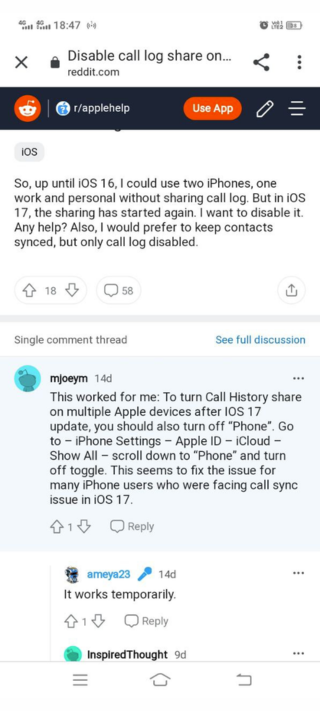**Detailed Caption:**

This screenshot showcases a Reddit conversation between users discussing a technical issue with iOS 17. At the top of the screen are various icons including an 'X', a lock symbol, a 'Disable' option, a 'Call' button, an activity log, and a 'Share on reddit.com' option. On the right-hand side, there is a three-dot menu icon situated above a triangular symbol with three horizontal dots. Below this, the Reddit logo and a black rectangular bar are visible.

The primary text in the screenshot reads: "So up until iOS 16, I could use two iPhones, one for work and one personal, without sharing the call log. But in iOS 17, the sharing has started again. I want to disable it. Any help? Also, I would prefer to keep contacts synced, but only disable the call log."

The response to this query suggests a solution: "This worked for me. To stop sharing call history on multiple Apple devices after the iOS 17 update, you should turn off the 'Phone' setting. Go to iPhone Settings > Apple ID > iCloud > Show All > Scroll down to Phone, and turn off the toggle. This seems to fix the issue for many iPhone users experiencing call sync issues with iOS 17."

A follow-up response reads, "It works temporarily."

Finally, there is a partially-cut-off reply from a user named "Inspired Thought."

Additional icons like a search bar labeled "Search for Apple help," a 'Use App' button, a pencil icon, and a three-line menu bar are also visible, suggesting various user interface elements of the Reddit app on an iOS device.